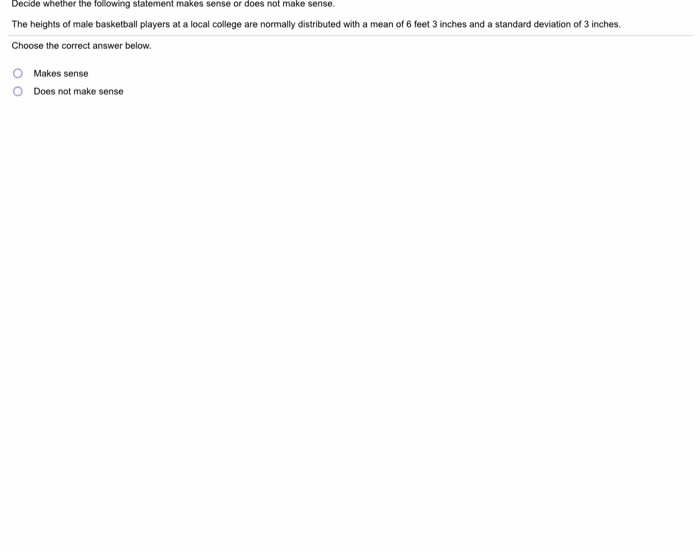A cropped screenshot displays a question from an online assessment. At the top left corner, in small black font, it reads: "Decide whether the following statement makes sense or does not make sense." 

Below this prompt, a question states: "The heights of male basketball players at a local college are normally distributed with a mean of 6 feet and 3 inches and a standard deviation of 3 inches."

A thin gray line separates the question from the answer options beneath it. Under the gray line, on the left side, the instruction "Choose the correct answer below" is printed. Two answer choices are listed vertically:

1. "Makes sense" with a clickable bubble to its left.
2. "Does not make sense" with a clickable bubble to its left.

Neither option is selected. All the text, including the question and answer choices, shares the same font style, color, and size.